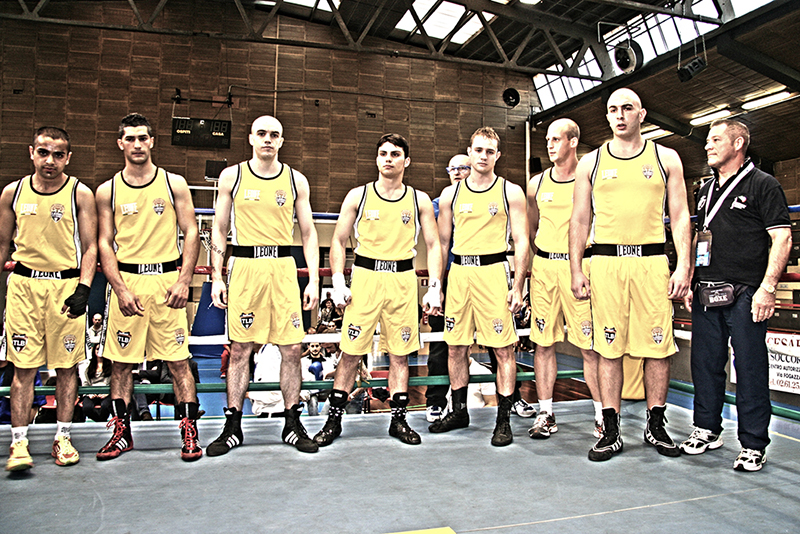The photo showcases a sports team of seven white men dressed in matching yellow tank tops and yellow shorts with black belts emblazoned with the letters "LEONE," standing inside a boxing ring. Their footwear varies, resembling wrestling shoes. Positioned to the right of the athletes is a man who appears to be the coach, distinguished by his black polo shirt, pink lanyard with a name tag, fanny pack, navy blue trousers, and sneakers. There is also a referee in the vicinity, wearing black pants and a blue shirt. The indoor setting features brown walls and skylights above, suggesting a gymnasium or sports facility. Additionally, other individuals are visible in the background, likely present for training purposes rather than as an audience. The team members are all looking directly at the camera.